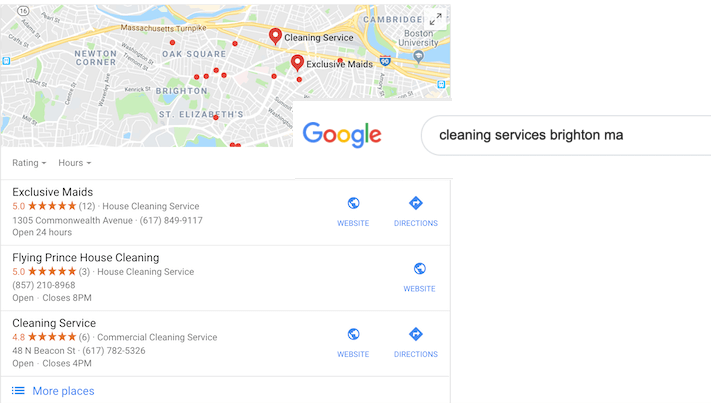**Detailed Caption:**

The image is a screenshot displaying the search results for "cleaning services Brighton MA." The background is predominantly white, with a minor overlay bar on the right-hand side partially obscuring the content. At the top of the screen, a map with multiple pins indicating various locations is visible, corresponding to the search results below.

Beneath the map, three primary search results are listed within a white box. The first result is for "Exclusive Maids," highlighted with a set of details including its perfect 5-star rating based on 12 reviews. This house cleaning service is located at 1305 Commonwealth Avenue, and its phone number is 617-849-9117. Notably, it is available 24 hours.

The second result is for "Flying Prince House Cleaning," which also boasts a 5-star rating. Although the phone number is provided, there is no accompanying address or directions available for this service.

The third result is simply titled "Cleaning Service," holding a 4.8-star rating from six reviews. This is a commercial cleaning service with both an address and a phone number provided. This service closes at 4 PM.

At the bottom of the search results, in blue text, the option to view "more places" is available for further exploration of cleaning services in the area.